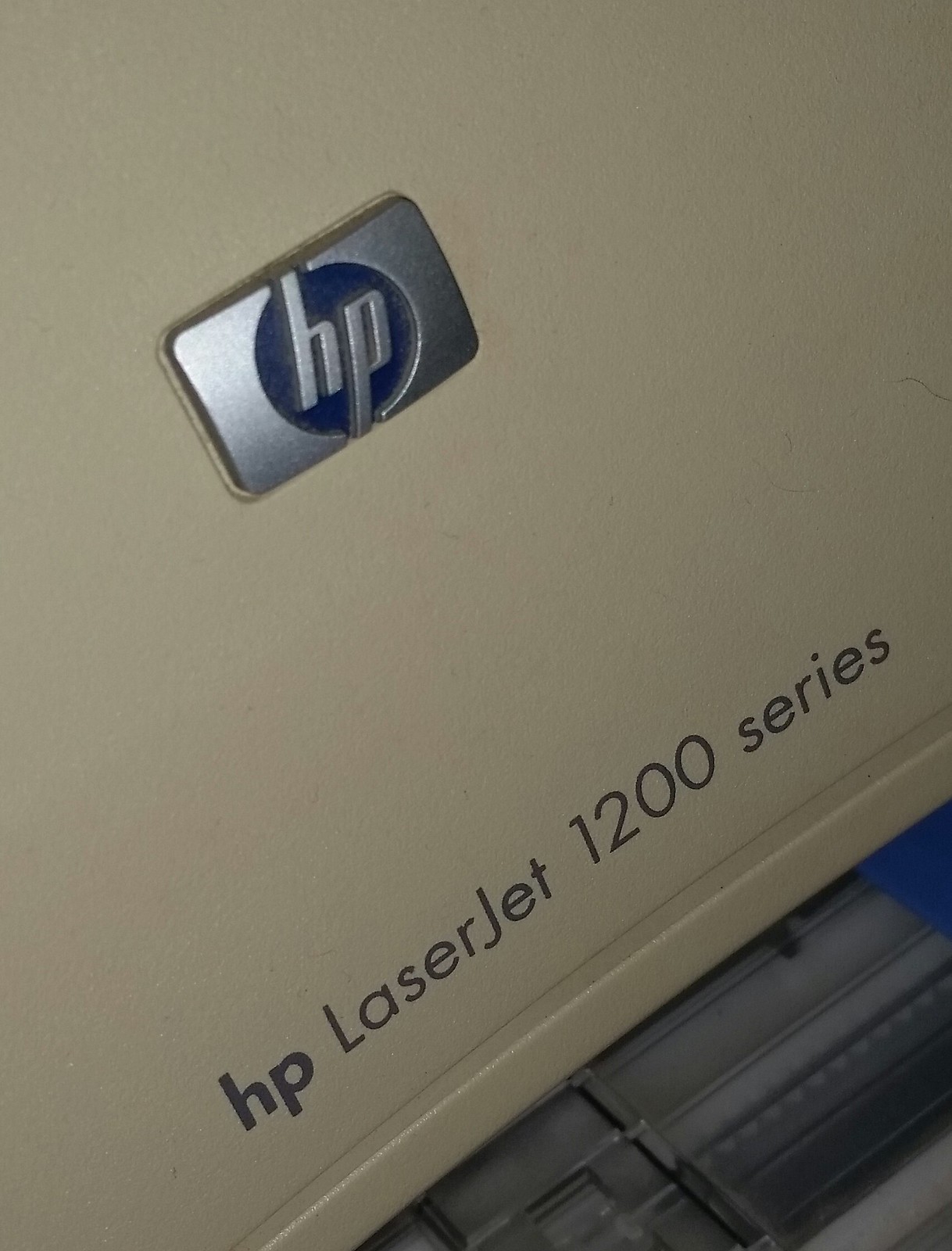The image presents an up-close shot of a printer, specifically the HP LaserJet 1200 series. The prominent feature in the photo is the HP logo, which consists of a metallic grey rectangle with a blue circle inside. Within this blue circle, the letters "hp" are displayed in metallic grey, lowercase. The printer body appears in an off-white or light brown color, often described as a biscuit color. Below the logo, the text "HP LaserJet 1200 series" is clearly visible. The photo is zoomed in to the point where additional features, like a small blue part and some black and green elements beneath the main text, are somewhat indistinguishable but may include a feeder tray or paper output tray. The close-up nature of the image makes it challenging to identify these parts precisely.